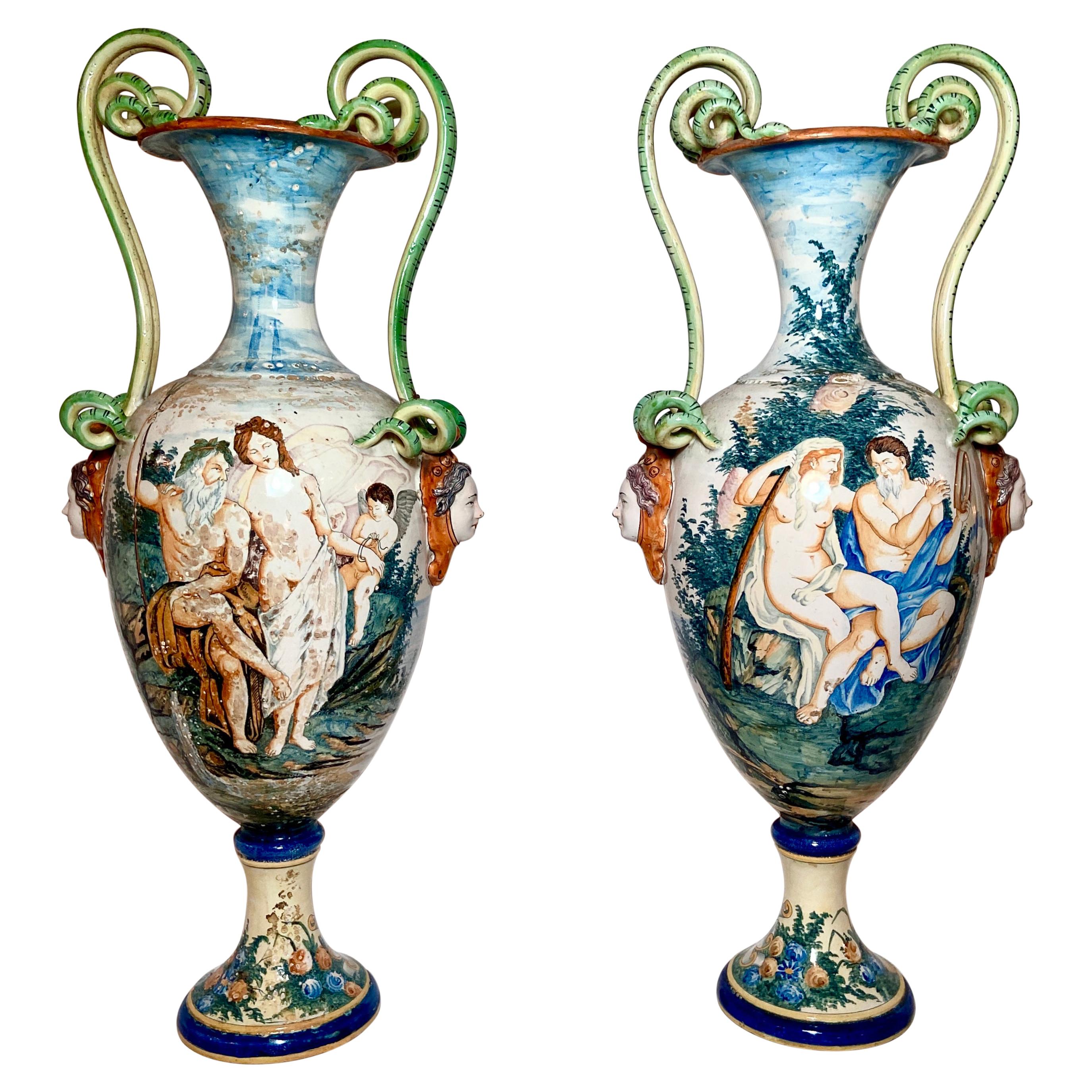The image depicts two ceramic vases, each intricately painted with detailed scenes that are reminiscent of 19th-century Greek art with a biblical nuance. Both vases are vertically oriented with oblong shapes that are bulkier in the center and taper off towards the tops and bottoms. 

The vase on the left features a central painting of a shirtless, bearded man sitting down, accompanied by a partially nude woman with red hair that cascades to her shoulders. A small, naked boy with black hair also appears in the painting, sitting amidst rocks and stones with a cloudy sky in the backdrop. Above the figures, green vines entwine near the top of the vase, and at the base, blue hues depict plants growing.

On the right vase, a predominantly blue and white background frames a similarly shirtless, middle-aged man with a gray beard and brown hair, wearing a blue cloth around his waist. Beside him sits a woman, also partially nude with red hair, swathed in white fabric around her lower half. The two figures appear to be in a conversation, surrounded by a serene setting of blue-green bushes and trees under a light blue and white sky.

Both vases have four snake-like handles—two per vase—painted in a light green color, ascending from the top and descending to the base. The vivid colors used across both vases include sky blue, white, orange, green, and beige, creating a rich, detailed scene that encapsulates a mixture of classical and religious aesthetics.